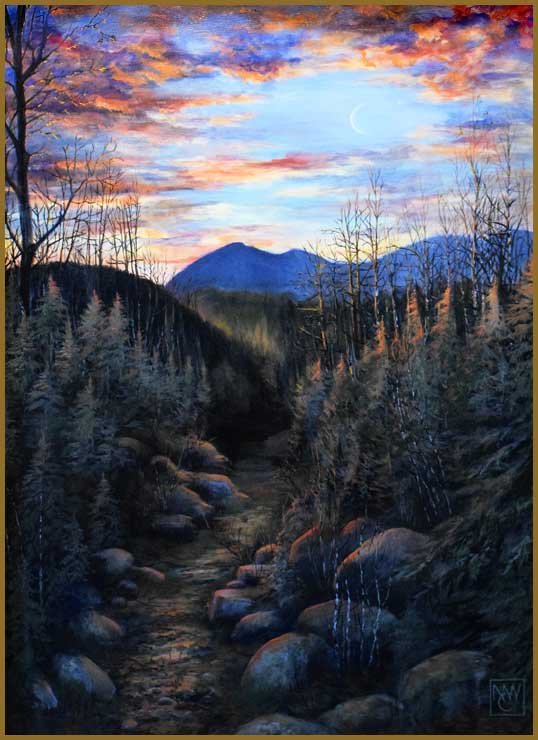The image depicts a stunning artist's rendition of a twilight forest scene set in the fall. The rectangular painting, approximately five inches high and four inches wide, is bordered by a thin one-eighth inch bronze or copper-colored outline. Dominating the top half of the picture is a dramatic sky, painted with light blue hues intermingled with dark orange and brown clouds, suggestive of an impending sunset. A delicate, thin white crescent moon peeks through an opening in the sky, enclosed by the vivid clouds.

In the distant background, a blue mountaintop range extends across the canvas, transitioning into dark gray hills as the eye moves downward. The foreground features large boulders flanking what appears to be either a narrow path or a dried-out stream bed, adding a sense of depth and intrigue. The hills are dotted with varied vegetation; barren, leafless trees, likely indicating late fall, and short pine trees interspersed with scrub oaks. One prominent, taller, leafless tree stands on the back left of the image, contributing to the seasonal feel of the painting.

The overall scene conveys a serene yet slightly melancholic ambiance, with the intricate details of the trees, rocks, and grasses adding to the realism that makes the painting almost photographic. The arrangement of natural elements guides the viewer's eye from the tranquil setting of the creek or path in the foreground, through the middle with its textured hills and sparse vegetation, to the majestic, looming mountains and ethereal twilight sky above.